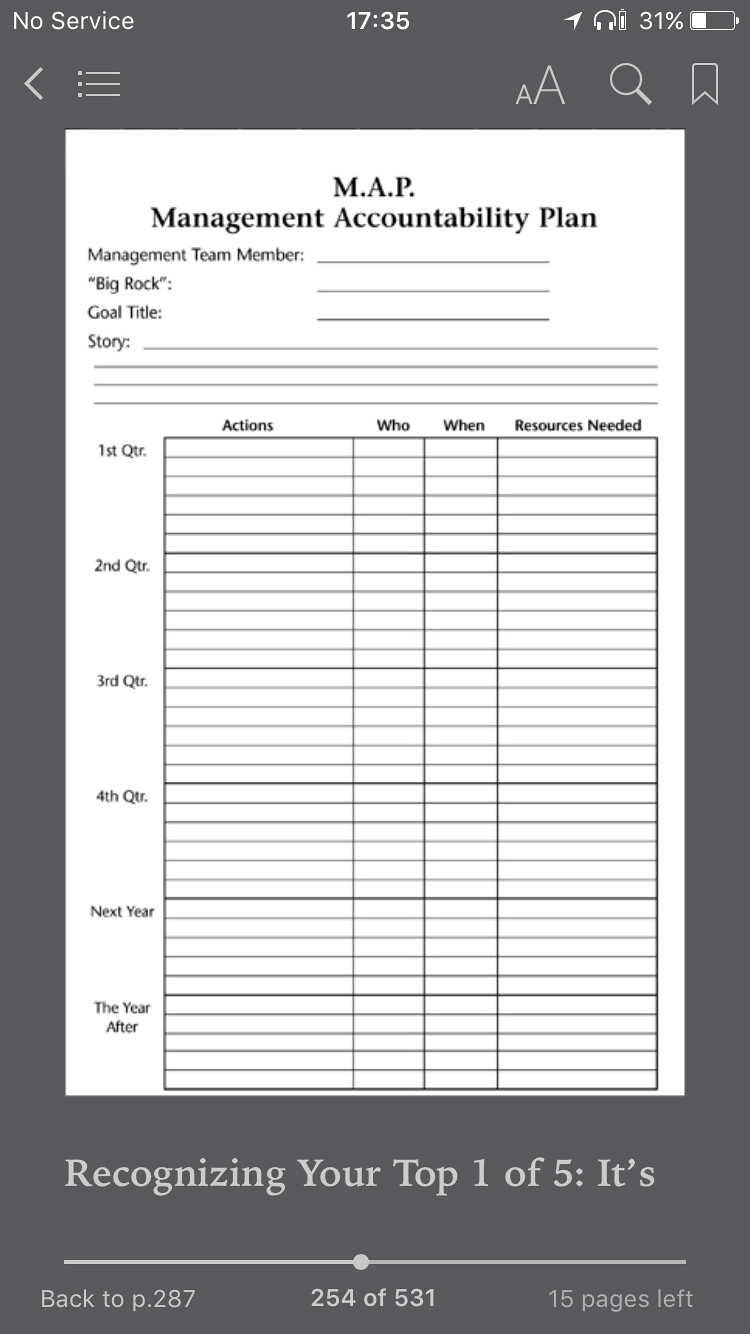This image is a screenshot of an iPhone screen displaying a document titled "MAP: Management Accountability Plan." The iPhone status bar at the top shows no service, the time as 7:35, and a 31% battery level. The interface includes back, menu, font adjustment, search, and bookmark buttons, all presented on a gray background. 

The document itself is a white page with a mix of red and black text and several lines meant for inputting information. Key sections include areas to fill out the management team number, Big Rock, and Goal Title. There are structured tables for entries under categories like "Actions," "Who," "When," and "Resources Needed" across various timeframes—first quarter, second quarter, third quarter, fourth quarter, next year, and the year after.

At the bottom of the screen, outside the document area, text reads "recognizing your top one of five," alongside a navigation bar indicating progress through the document, showing "back to page 287," "255 of 531," and "15 pages left." The overall layout suggests a detailed plan for management accountability with multiple areas for detailed inputs and tracking progress over time.